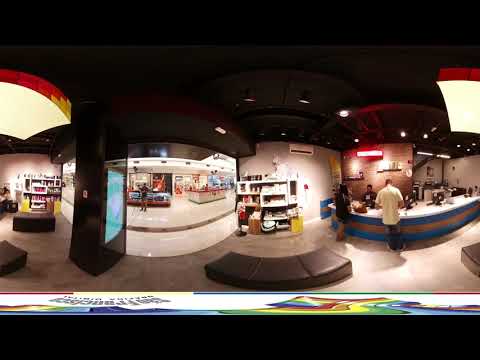The photograph captures an interior view of a bustling mall, focusing on a specific store situated within it. The mall's floor is a tan color, and the hallway walls are decorated with various colors, creating a vibrant atmosphere. Dominating the center of the image is a curved, brown cushioned bench, which offers seating for visitors. On the right side, there is a service counter with a blue and gold circular design, illuminated by red lighting from the store behind it. This store appears to be an ice cream or candy shop, evidenced by cake-like items displayed on shelves to the left. Several people are visible in the scene: a cashier assisting three women, one of whom is purchasing a brown box, and a man in a yellow shirt who seems to be preparing to make a purchase. Additionally, a black pillar with blue detailing can be seen, adding to the mall's aesthetic. An LCD screen kiosk is also visible on the left side, displaying visual content to passersby. Overall, the photo effectively captures the lively and colorful ambiance of a mall environment.